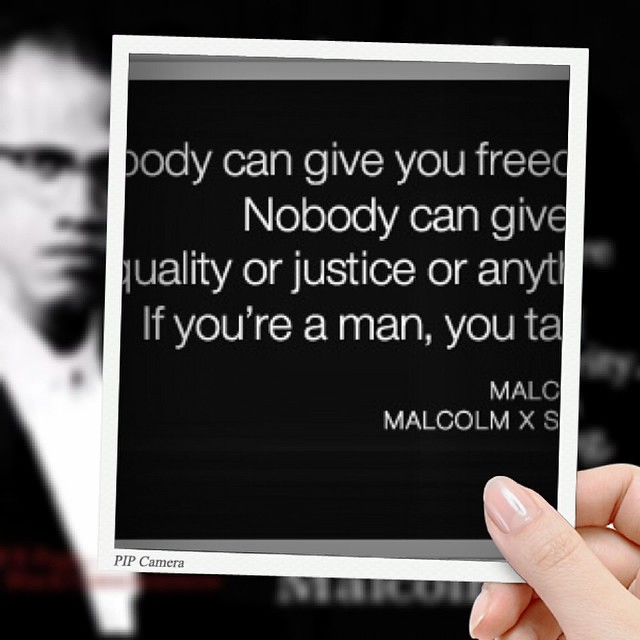A woman with clear, glossy nail polish holds up a black card with white text. The card features a partially visible quote: "Nobody can give you freedom, nobody can give you equality or justice or anything. If you're a man..." The rest of the quote is obscured. The signature "Malcolm X" is at the bottom of the card. In the background on the left side, a somewhat blurred black-and-white photograph of Malcolm X is visible. He is wearing horn-rimmed glasses, a white button-down shirt, and a jacket. His image adds context and depth to the message being held in the foreground.